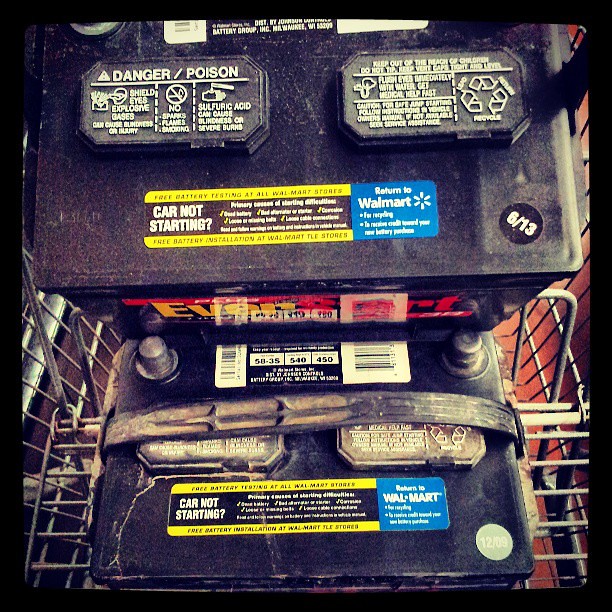This overhead photo showcases two old, slightly dusty car batteries placed in the child seat section of a shopping cart. The batteries feature a prominent blue rectangular sticker with white text, indicating "return to Walmart." Each battery also displays another sticker with a yellow border on the top and bottom, and a black center section with white lettering that reads "Car not starting?" Additionally, there are informative labels on both batteries, including one displaying a warning marked "danger/poison." The battery positioned on top has a date sticker reading "6/13," while the one underneath has a less legible date sticker that appears to show "12/09." The shopping cart's design allows the reddish floor to be visible through its metal frame, further emphasizing that the batteries are likely en route for troubleshooting or return.